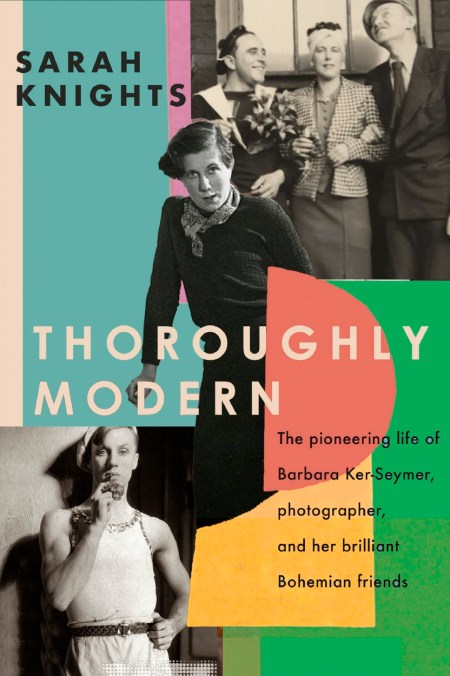This image appears to be the cover of a book, designed in a vertically rectangular format with an eclectic blend of colors and geometric shapes. The background features a complex arrangement of color blocks: a light tan stripe runs vertically on the upper left, merging into areas of blue and light purple, while the bottom showcases green. A prominent red sideways arch is positioned just right of center, beneath which begins a yellow rectangle progressing diagonally from top right to center left. 

Three black and white photographs adorn the cover. In the top right corner, an image captures two men, possibly in drag—the left one in a sailor suit, the one in the middle holding flowers and a wine glass, and a third figure, a man in a cap and suit, looking upward. At the center, a different woman is depicted wearing a scarf around her neck with a black sweater and skirt. Lastly, the bottom left features another person, wearing a sleeveless shirt, belt, and pants, possibly holding a cigar.

The text on the cover includes prominent titles and information: "Sarah Knight's" in black capital letters at the top left corner, "Thoroughly Modern" in white capital letters across the middle, and "The Pioneering Life of Barbara Kerr Seymour, Photographer and Her Brilliant Bohemian Friends" in the lower right corner. The cover’s dynamic layout and vivid details emphasize the subject's pioneering artistic community and eclectic bohemian lifestyle.